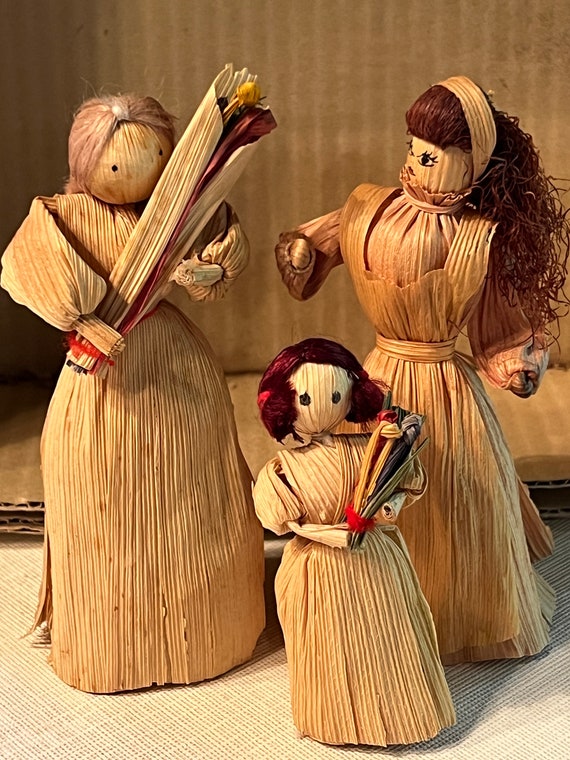The image features a trio of corn husk dolls, set against a backdrop of a cardboard box turned on its side, revealing its vertical brown lines. The base or floor is a light tan canvas-like surface with a fibrous cross-hatch design. The dolls are intricately detailed and represent an older woman, a younger woman, and a little girl.

The older woman, positioned on the left, has light pink yarn hair parted down the center and small black beady eyes. She is clad in a dress and holds a long bouquet with a small yellow flower. Her hair appears to be made from some coarse fiber or thick paper. 

The younger woman on the right has long, curled dark brown hair, possibly made from a material other than yarn. She wears a dress with a headband and has a strikingly mean-looking face with larger, drawn-on eyes complete with eyelashes and red lips. 

In the center front is the little girl, distinguished by her short velvety red hair. She also wears a dress and holds a small bouquet featuring blue, yellow, and red flowers. Her face is simple, with two large circular eyes.

The detailed craftsmanship of the corn husk dolls, combined with their distinctive features and attire, create a captivating, homely scene enhanced by the rustic cardboard background.